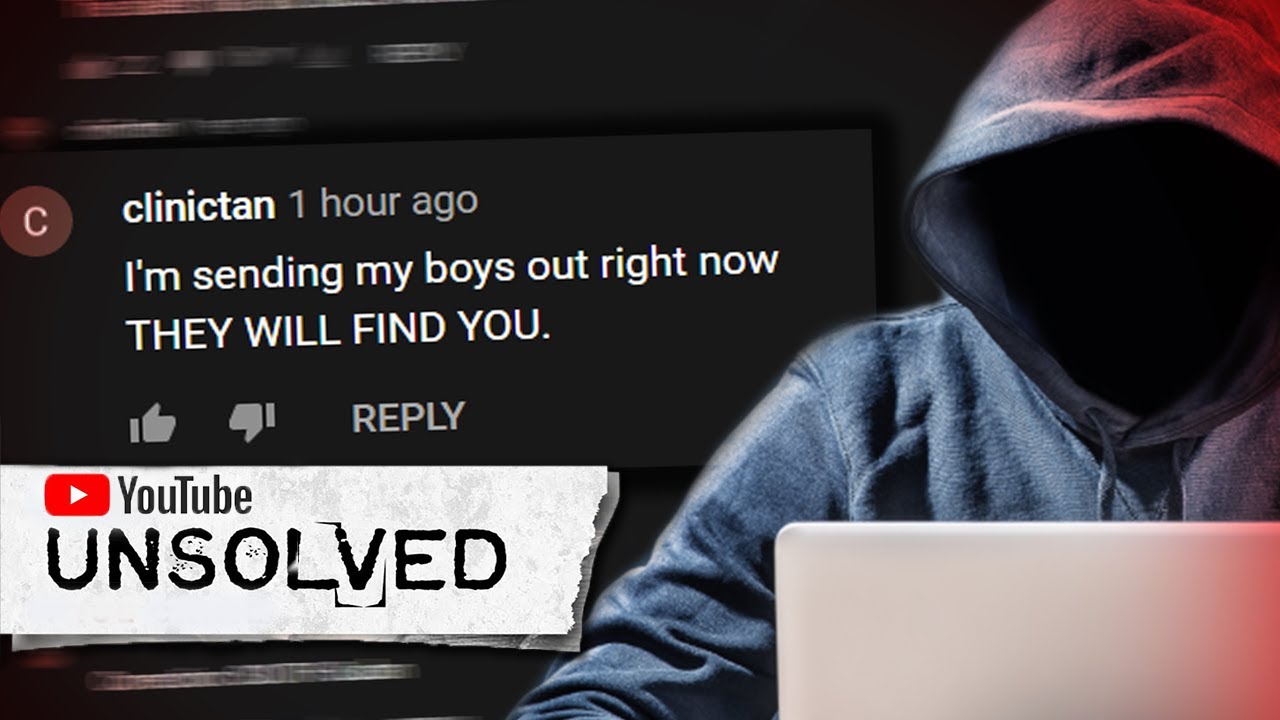The image depicts a YouTube thumbnail for a video from the channel "YouTube Unsolved." The thumbnail is dark and mysterious, featuring a hooded figure whose face is obscured by shadows. The person is seated in front of a PC, depicted on the right side of the image. On the left side, there's a comment icon indicating engagement. 

Overlaid text includes a recent comment from a user named Clinton, timestamped one hour ago. The comment reads, "I'm sending my boys out right now. They will find you," emphasized in bold letters, suggesting a threatening tone. Below this comment, standard YouTube interaction buttons such as like, dislike, and reply are visible.

At the bottom of the thumbnail, the YouTube logo is prominently displayed with the familiar red play button icon that includes a white triangle in the center. The text "YouTube unsolved" is also visible, identifying the possibly eerie, investigative nature of the channel.